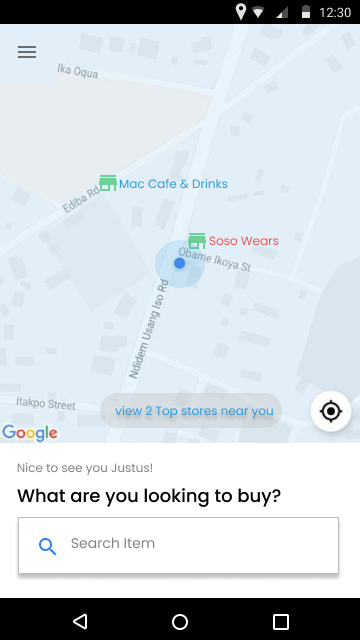This is a detailed screenshot from a mobile device, most likely a smartphone, showcasing a map view within an unfamiliar app. The top 5% of the screen is a black header bar featuring white icons, including a location pin, Wi-Fi signal strength, cellular signal strength, battery indicator, and the time, which reads 12:30.

Below the header, about three-quarters of the screen is occupied by a map view with several roads. The roads are labeled in Roman characters, but not in English. Key streets include Ika Opa, running east to west; Ediba Road, running southwest to northeast; and Didem Usang Iso Road, running north-south. The user’s location is marked by a blue dot at the intersection of Didem Usang Iso Road and Obama Ikoya Street, indicating the GPS position and its accuracy range. 

Another road, Itako Street, runs east-west further south. Notable points on the map include green shop icons. Across from the blue dot on Obama Ikoya Street, a shop labeled "Soso Wares" appears in red text. Another shop labeled "Mac Cafe and Drinks" on Ediba Road is marked with blue text. The bottom-right corner of the map view shows the Google logo in its iconic colors, while the bottom-left corner features a target locator icon. Between these, a blue-text link in a gray bubble invites the user to "view two top stores near you."

The lower section of the image features black text on a white background, greeting the user with "Nice to see you Justice," followed by a bold, larger text asking, "What are you looking to buy?" This section includes a blue magnifying glass icon within a search box. The bottom footer displays the typical Android navigation buttons: back, home, and the "apps open" button, all in white on a black background.